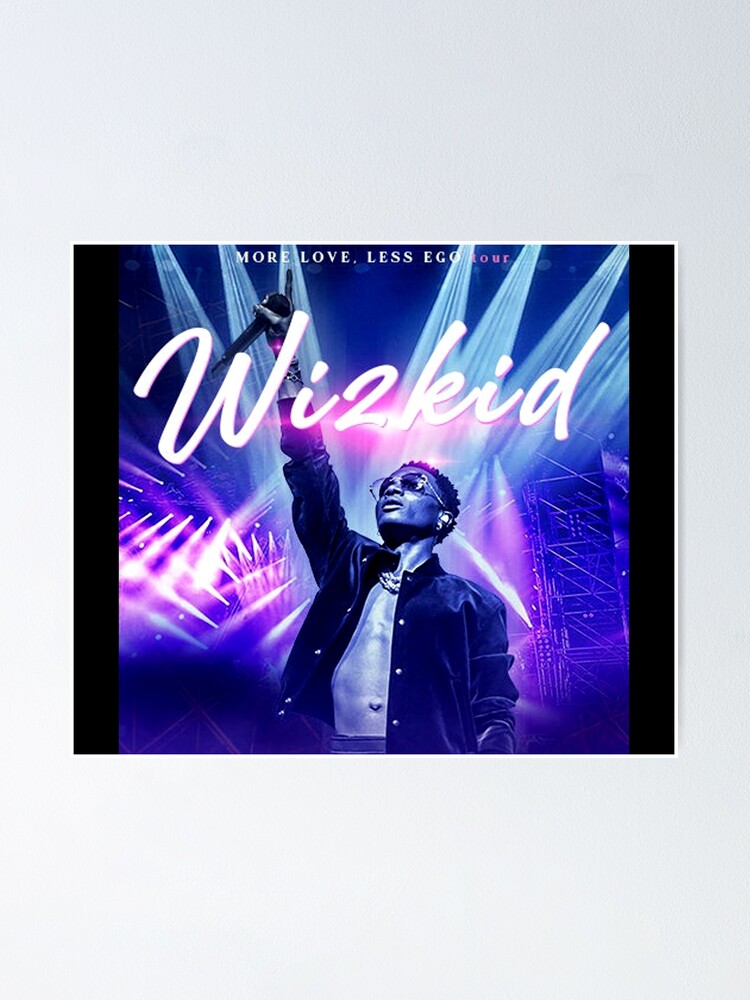The image is a color photograph in landscape orientation, designed as a CD cover or jacket. Centered in the image is an African-American male, identified as WizKid, wearing an open dark-colored jacket with no shirt underneath, two necklaces, and black sunglasses. He has short dreadlocks and a focused, upward gaze toward the left side of the image. The man holds a microphone in his right hand, which is raised above his head, with his index finger pointing skyward. Text in white at the top of the image reads "More Love. Less Ego. Tour" in bold script, and directly below this, above the man's head, is the name "WizKid." The background features an array of spotlights—blue at the top and purple at the bottom—illuminating the scene, with a fretwork of metal visible on the right side. The image is bordered by thin black bars on the left and right, giving it an appearance suggestive of both a CD art cover and a poster. The overall style combines photographic realism with graphic design elements.